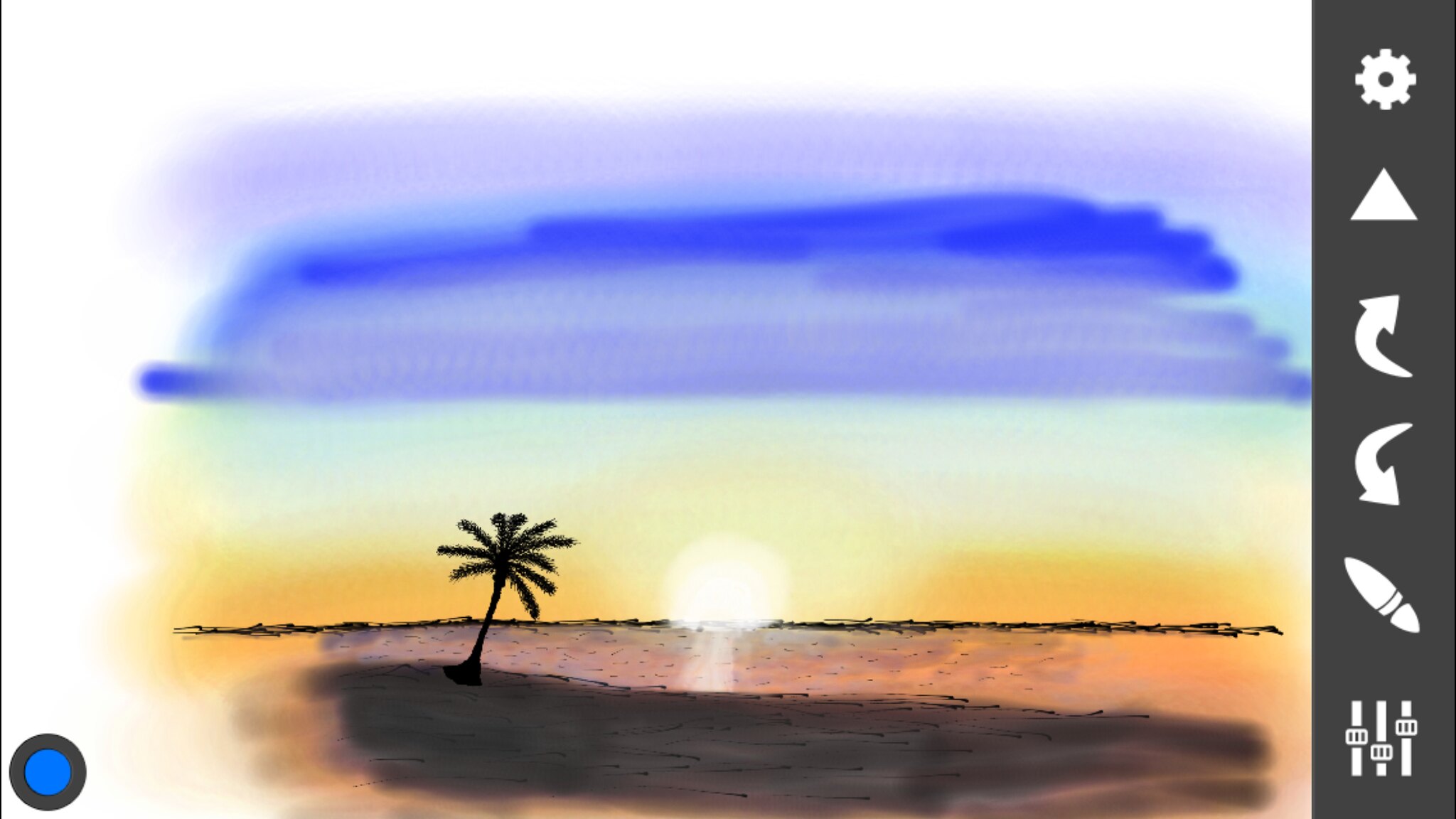This screen capture showcases a digital art application featuring a detailed digital painting of a sunset. The interface includes a horizontally aligned rectangle with a vertical gray toolbar on the right side, adorned with white icons for settings, undo and redo buttons, a paintbrush, and three adjustable dials. In the lower left corner is a small blue circle outlined in gray, likely an editing tool.

At the center, the main canvas depicts a striking sunset scene. The sky transitions from white at the very top to blue, gradually blending into orange and yellow near the horizon, capturing the essence of dusk. Below the vibrant sky, a stark black line outlines the horizon just above the setting sun. The foreground presents gray land, possibly representing a beach or desert, with very dark shadows adding depth to the scene. To the left, a black silhouette of a palm tree stretches upwards, its leaves partially extending into the circular editing tool on the bottom left. This intricate artwork, seemingly created with markers or digital brushes, highlights the blending of colors and shadows, emphasizing the serene yet vivid atmosphere of a sunset.